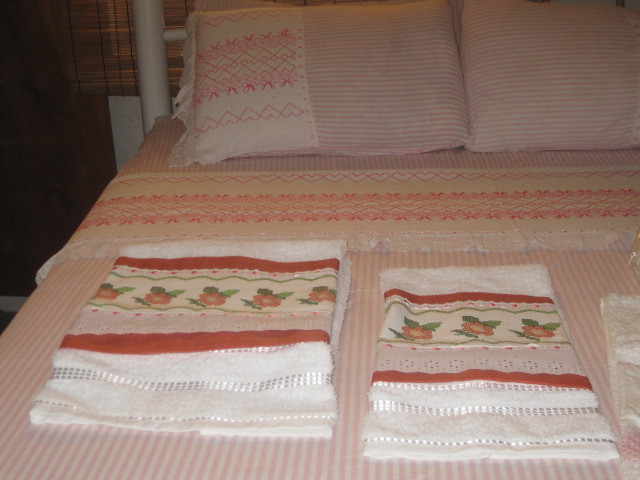In this detailed photograph of a bedroom, the focus is on a meticulously arranged double bed with a white metal frame. The bedspread showcases a combination of pink and white stripes, complemented by pillowcases featuring both stripes and intricate cross-stitched patterns with pink hearts lined neatly. At the headboard, you notice its white pole construction with delicate bands.

Toward the front of the bed, there are two types of towels neatly folded: one set showcases a design of reddish-orange flowers with green leaves, set against a white background with stripes, while another set features a quilted embroidery with roses on a white background. The towels appear newer and brighter compared to the bedspread, and they include both a bath towel and a hand towel, each adorned with lace detailing.

The bedroom itself contains a brown door and white-painted wall partially visible in the background, accompanied by old-fashioned, orange-and-red plaid curtains. The photo was taken indoors with a flash, emphasizing the bed and the distinct patterns and textures of the linens while casting some areas into shadow, such as a nearby cabinet.